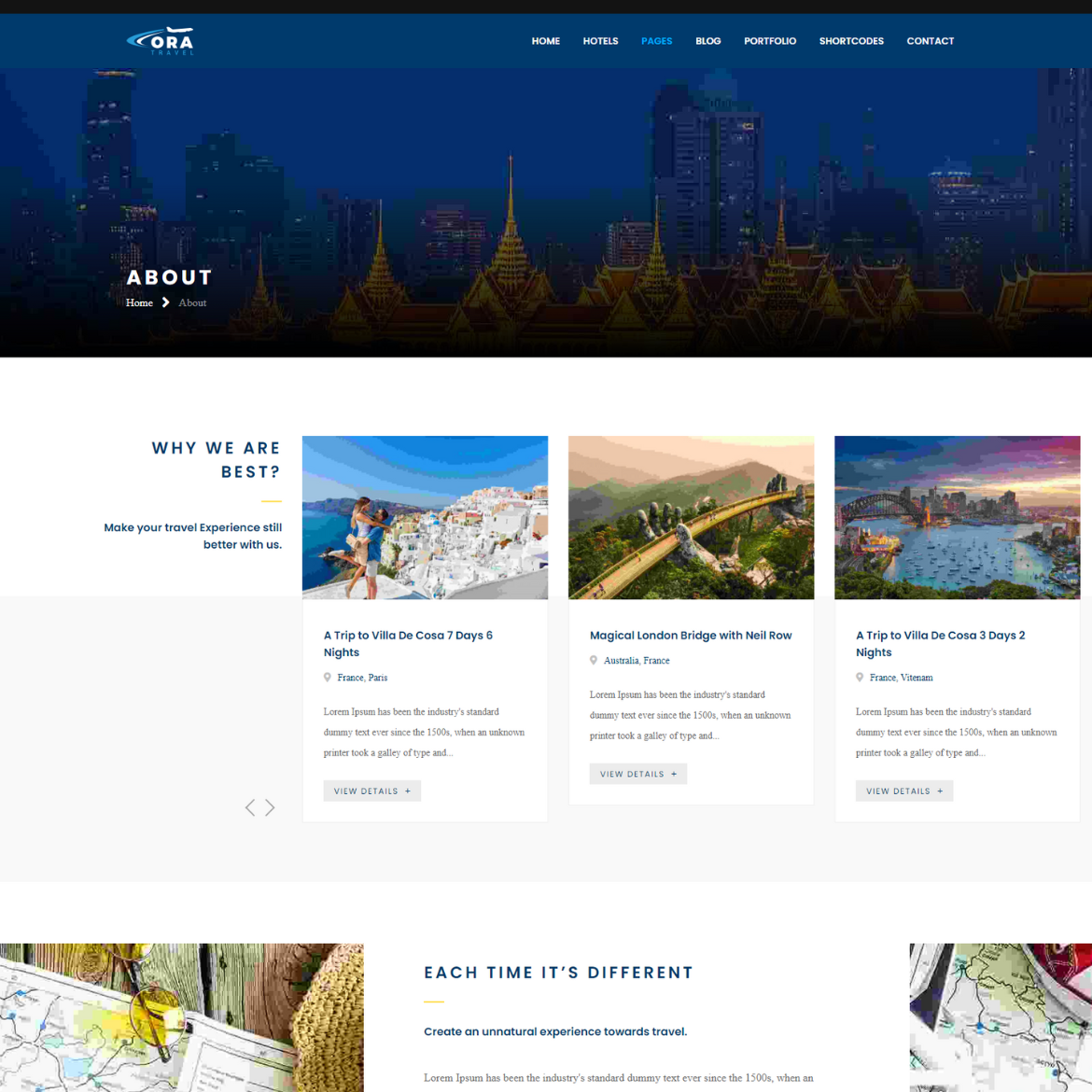On the travel company's website "Ora" (spelled O-R-A), visitors are greeted with a cityscape at night, providing a captivating backdrop for the menu bar at the top of the page. The menu includes options for Home, Hotels, Pages, Blog, Portfolio, Short Cooks, and Contact. The current page being viewed is the "About" page.

Centered beneath the menu, a striking tagline in blue lettering reads, "Why are we the best? Make your travel experience even better with us." Below this, the website showcases three example tours, each accompanied by an evocative image.

The first tour is a seven-day, six-night trip to "Villa da Cosa" in France, specifically listing Paris, although the title might be confusing. The accompanying image features two individuals in swimsuits and towels, relaxing at a beach resort, with pristine white buildings and the deep blue ocean providing a picturesque backdrop.

The second tour advertised is titled "Magical London Bridge with Neil Rowe" and mentions Anatolia in France inaccurately. The photo features an impressive pedestrian walkway supported by two enormous stone hands, with green-roofed mountains stretching out behind them, creating a surreal and enchanting scene.

The third offering lists another trip to "Villa da Cosa," this one lasting three days and two nights. The photograph shows a tranquil bay with a large bridge extending across it, accompanied by the distant cityscape in the background, enhancing the sense of an inviting destination.

Overall, the site elegantly presents its array of tours, enticing potential travelers with stunning visuals and compelling narratives.